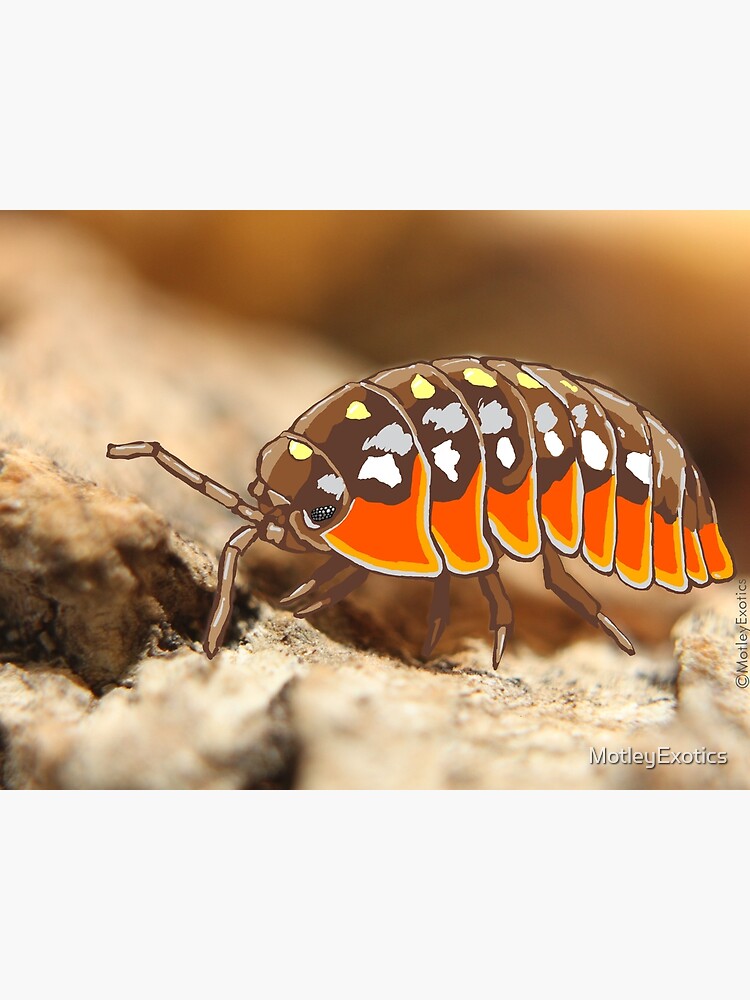In this detailed image, we see a digitally illustrated, beetle-like bug superimposed on a real photograph of a rocky ground. The vibrant creature features a hard shell with a striking color palette, reminiscent of a monarch butterfly. Its back is primarily brown adorned with numerous yellow and white spots, while the sides are orange, bordered with thin stripes of yellow and white. The beetle's dark brown legs, of which five are visible, extend across the image. The antennae are raised, adding to the lifelike appearance. The rocky background beneath the bug is composed of brown and black hues, creating a stark contrast with the vivid colors of the insect. The image credits "Motley Exotics" in white print at the lower right corner, indicating its creator.